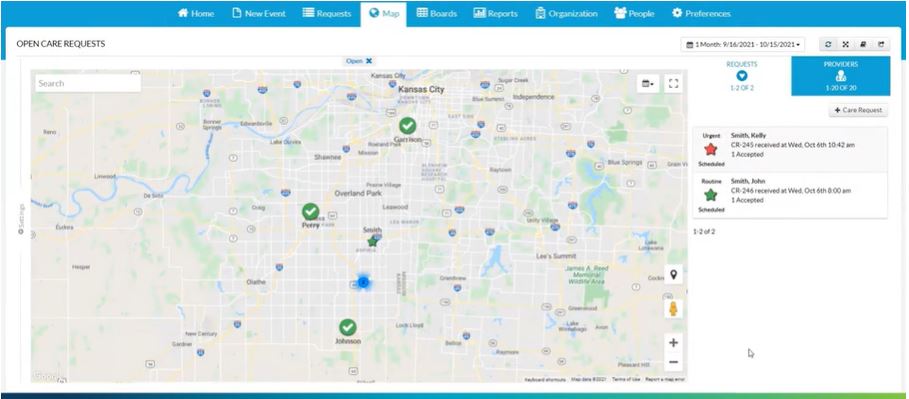This detailed caption describes a horizontally oriented color screenshot of a user interface. The image has a white background and is dominated on the left by a large, detailed map of Kansas City, which occupies the majority of the space. The right-hand side features a control panel with a vertical list of buttons corresponding to different sections of the interface: Home, New Event, Requests, Map, Boards, Reports, Organization, People, and Preferences. 

The "Map" tab is highlighted, identified by a globe icon. Directly beneath it, the label "Open Care Requests" is visible. The map displays highways with labeled interstate icons and marks three locations of interest with checkmark icons. At the top right of the map, there is an icon for expanding the map view. The lower right corner includes Google Maps icons such as a location pin, a street view icon, and zoom in/out buttons.

On the right side of the interface, the top section features a dropdown menu labeled "one month, 9-16-21 to 10-15-21" for selecting date ranges, accompanied by various filter and sort icons. Below this, a blue box displays the number of requests and provinces or providers. The names of two providers are listed underneath: Smith Kelly and Smith John, each marked by a distinct star icon (red and green, respectively). The green star is pinpointed on the central part of the map, indicating a specific location.